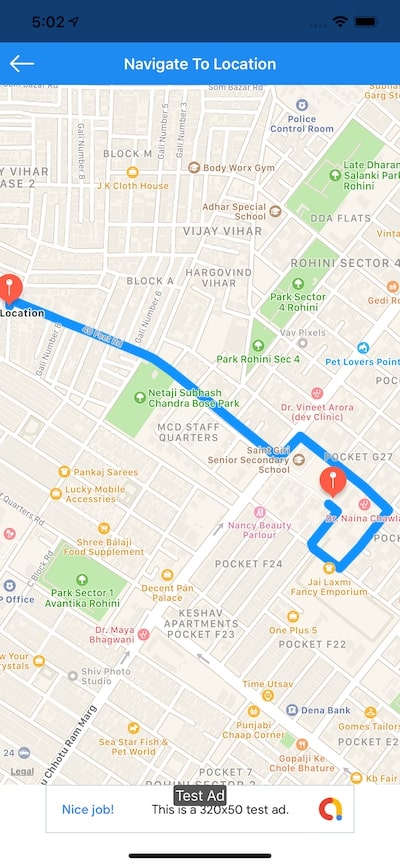The image features a blue-themed user interface with various navigation elements. The background is a gradient of blue, with a dark blue strip at the top right corner containing two small black icons resembling an arrow and a battery indicator. Below this strip, a lighter blue box displays a white left arrow accompanied by the text "Navigate to Location."

The main portion of the image is dominated by a map displaying a neighborhood. On the map, a red tag labeled "Location" marks a point of interest, while a prominent blue line traces a route back to a starting point marked by a red pin.

At the bottom of the image, there is a black box containing the text "Test Ad" beside a white drop-down box with the phrase "Nice job." Below this section, a colored semicircle with shades of blue, yellow, orange, and red is featured, followed by a thin black line that runs horizontally across the bottom of the image.